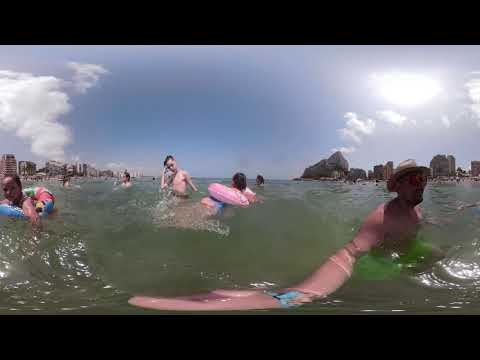This image captures a lively scene of people enjoying a day in the water, likely in the ocean or possibly a lake given the ambiguity and low image quality. The centerpiece of the photo is a man on the right side, his hand raised toward the camera. He sports sunglasses and a hat, with lime green swim trunks visible through the water. Surrounding him, in the central part of the image, are several children. One child is inside a pink inner tube, while another stands nearby. To the left, a young girl floats in a multi-colored inner tube featuring blue, red, green, yellow, and perhaps white. Additional people are present in the blurred background, with some distant buildings visible to the right and left edges. The sky is mostly clear with a few clouds, partially obscuring the sun in the top right corner. Despite the blurriness and potential VR distortion, the image suggests a clear day and captures the essence of a fun day at the beach or lake.